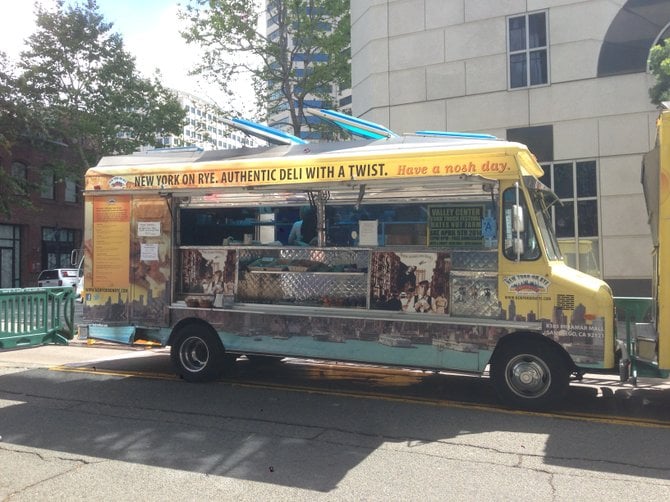In the image, there is a distinctive yellow food truck that resembles a converted school bus with vibrant and detailed artistry. The side of the bus prominently displays the text, "New York on Rye: Authentic Deli with a Twist. Have a Nosh Day." Above the bus, there are fins colored blue and white. The windows are open, and trays or other serving equipment are visible.

The exterior of the bus is adorned with various paintings and photographs. There's an image near the wheels that depicts a body of water with what could be ships or structures in it. Another photo on the side shows several people with the iconic figure of King Kong in the background. Alongside, text that may include a menu accompanies these visuals, though some parts are difficult to read. Additional signage around the bus includes "Valley Center," "Bates New Farm," and other unclear text.

The food truck is parked on a city street, surrounded by other vehicles and green fencing. In the background, city buildings, including a structure made of white limestone blocks, can be seen. This scene intricately blends urban and artistic elements, providing a unique and eye-catching visual experience.